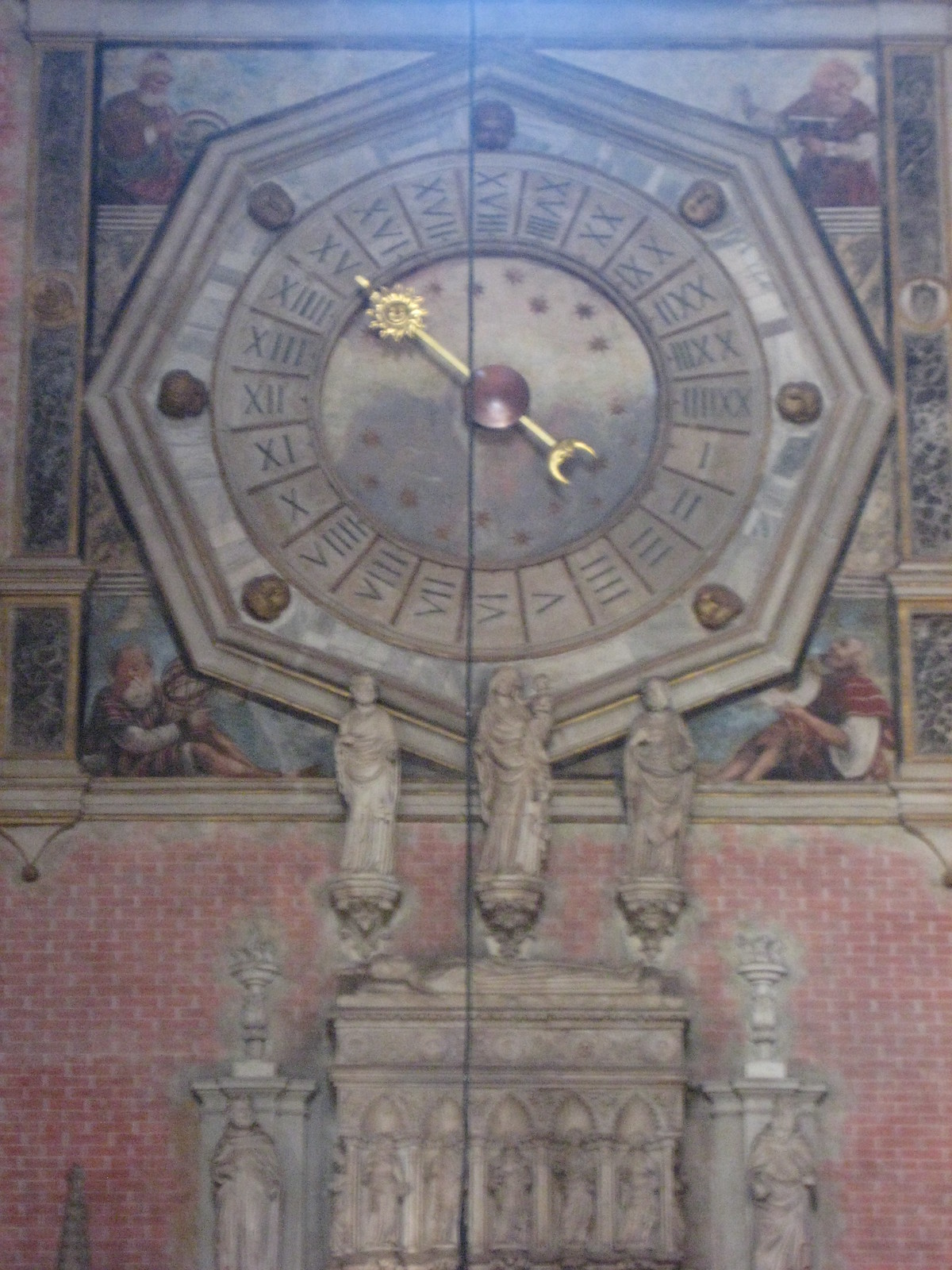This detailed image captures a close-up of a richly decorated fresco painted on the side of a building. Dominating the scene is a large, hexagonal clock with a gray face, embellished with splotches of blue. Within this hexagonal shape are seven gold-accented circles. Encircling these, the clock face features black Roman numerals and finely detailed hash marks, along with a maroon circle at the center where the clock arm pivots. The clock arm itself is striking, gilded in gold, with a crescent moon shape at the end and a small, sun-like circle also in gold on the opposite end.

Surrounding the central clock are intricate murals incorporating individuals dressed in brown, red, and green clothing, positioned at the top left, top right, bottom, and right sections of the fresco. Beneath the clock, a red brick wall forms the foundation, adorned with three statues of individuals in light gray—one of which appears to be the Virgin Mary—flanked by more statues on the left and right. Additionally, a parthenon-like structure, rendered in light gray and light brown, is placed prominently in the middle of the bottom section of the fresco, enhancing the historic and artistic ambiance of the entire scene.